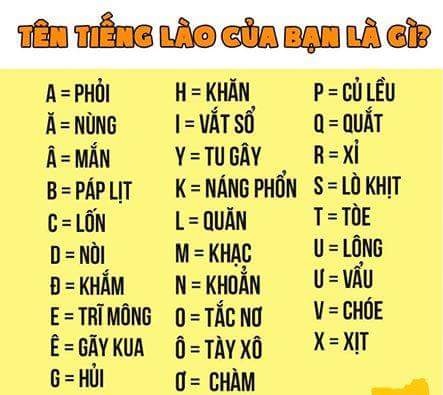The image is an educational infographic likely focused on the Vietnamese alphabet, though it could be another Southeast Asian language. The display has a yellow background with both orange and black text. At the top, there is a phrase written in orange font, "Tên Tiên Lào Quảng Bàn Lào Ghi?" Below that, the alphabet is presented using Latin letters. Some characters have diacritic marks such as accents or a "carrot" symbol. The letters displayed include multiple versions of A, D, E, and O, as well as single occurrences of other letters: B, C, G, H, I, Y, K, L, M, N, P, Q, R, S, T, U, V, and X. Next to each letter is an example word showing its pronunciation or usage, suggesting the infographic is designed to teach the pronunciation of these letters in both the native language and English.